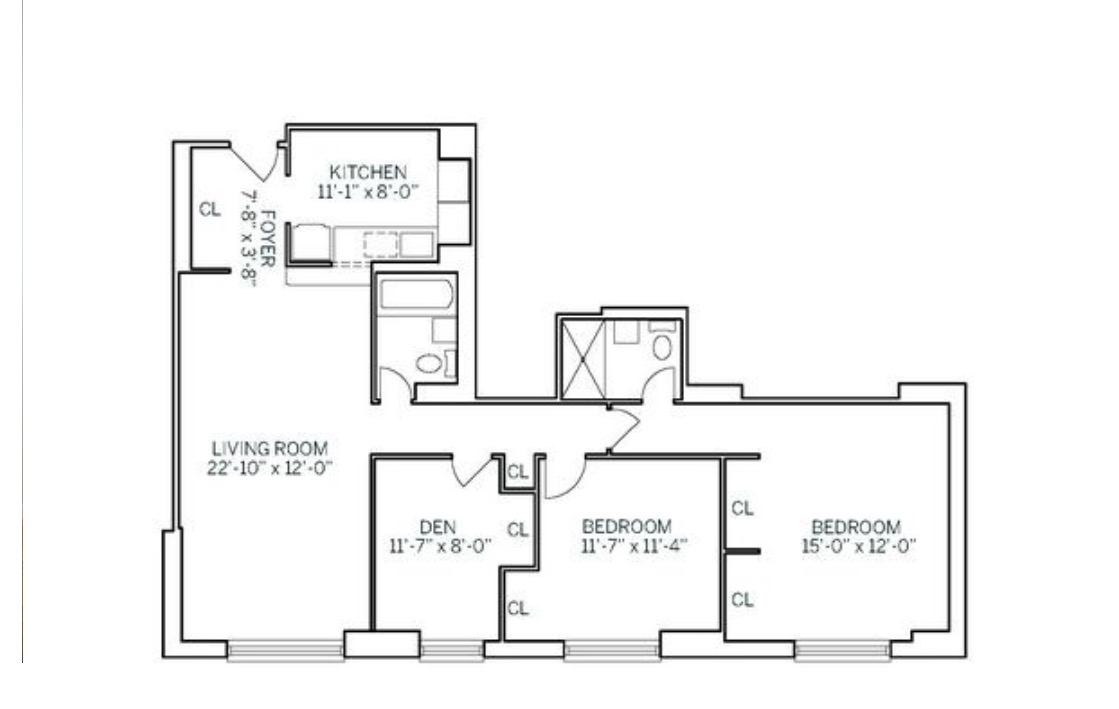The blueprint, set against a white background, intricately details the floor plan of a house. Rendered in black ink with supplemental light blue ink highlighting key elements, the design provides a clear and precise layout.

The living room, spacious and inviting, measures 22 feet by 22 feet 10 inches by 12 feet, marking it as a substantial and adaptable area. Adjacent to it is a foyer spanning 7 feet 8 inches by 3 feet 8 inches, featuring a door that opens into this welcoming space.

Off the foyer lies the kitchen, an 11 feet 1 inch by 8 feet area, thoughtfully designed to accommodate the sink and various appliances, thus ensuring a functional and efficient workspace.

A conveniently located bathroom sits between the living room and the kitchen, offering easy access from both areas. The den, positioned nearby, measures 11 feet 7 inches by 8 feet and includes a handy closet for storage.

A hallway leads to a half bath, situated for practicality, and directly across from it is a bedroom measuring 11 feet 7 inches by 11 feet. Finally, the floor plan culminates in a generous master bedroom, measuring 15 feet by 12 feet, complete with two large closets, providing ample storage and space for relaxation.